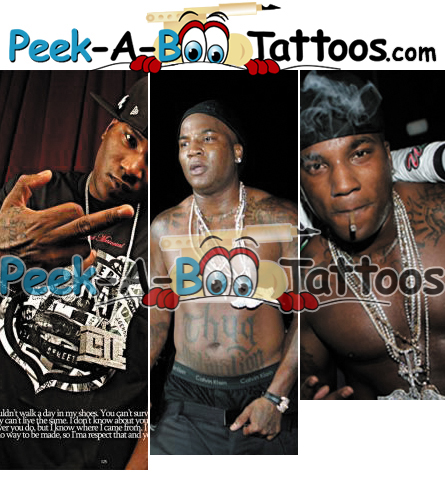The image is from PeekabooTattoos.com and features three men each in their own grid section, set against a white bordered top. All three men are black, heavily tattooed, and wearing distinctive accessories.

**Left Section:** A man in a black t-shirt and black box hat is flipping off the camera. His head is tilted sideways. There is partial white text under him that reads "walk a day in my shoes you can't can't live the same I don’t know about you you do but I know where I came from way to be made so I’m a respect that."

**Middle Section:** A shirtless man is adorned with numerous tattoos covering his stomach. He's decked out in multiple chains around his neck and is wearing a black hat-like fishnet on his head. The word "boo" is displayed in front of him, with the O's replaced by blue eyes.

**Right Section:** Another man with slicked-back black hair is seen with a dark cigarette in his mouth. Sporting a tattoo on his shoulders, he also wears a black hat and silver chains around his neck.